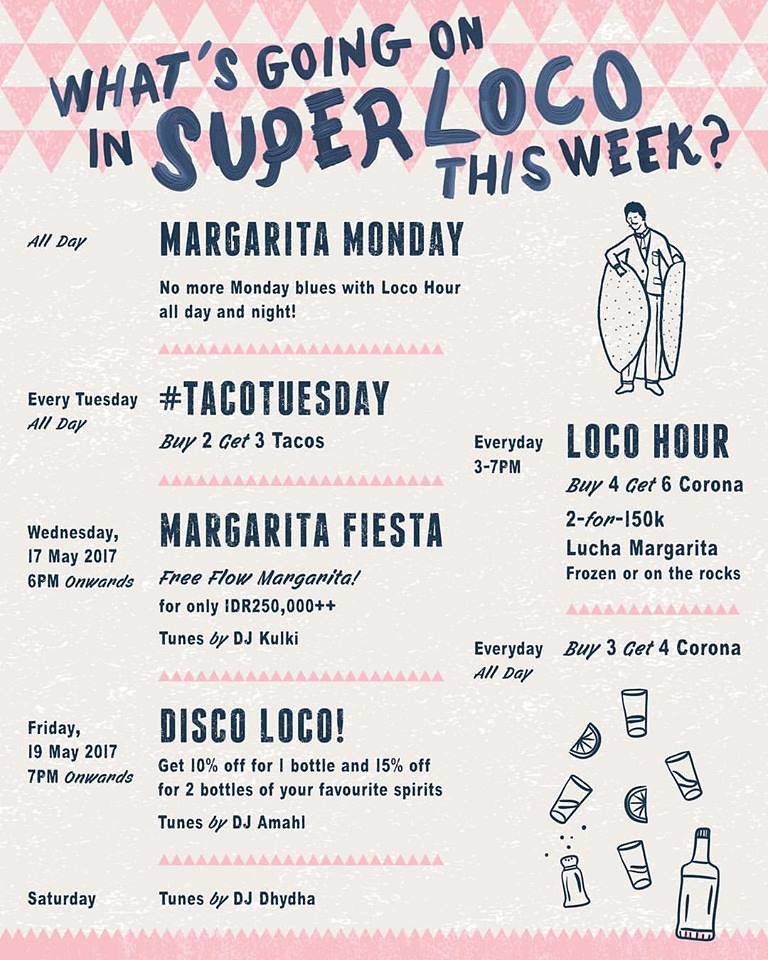The image is a detailed event schedule for the week at Super Loco, a restaurant or bar. The background is grey, adorned with various pink lines, triangles, and designs, creating a lively atmosphere. The text is written in a dark blue, casual, almost painted style. The headline reads, "What's going on in Super Loco this week?"

- **Margarita Monday (All Day):** Start your week right with "Loco Hour" running all day and night to keep those Monday blues away.
- **Taco Tuesday (All Day):** Enjoy Taco Tuesday with a special offer—buy two, get three tacos.
- **Margarita Fiesta (Wednesday, May 17th, 2017, 6 PM Onwards):** Indulge in a free flow of margaritas for only IDR 250,000++. Tunes by DJ Kulky.
- **Disco Loco (Friday, May 19th, 2017, 7 PM Onwards):** Dance the night away with 10% off one bottle and 15% off two bottles of your favorite spirits.

The design elements also include drawings of a man wrapped in a tortilla, drinks, shot glasses, and liquor bottles. The schedule offers additional deals like "Loco Hour" daily from 3 to 7 PM, with promotions such as buy 4 get 6 Coronas for 150K and Lucha Margaritas, either frozen or on the rocks.